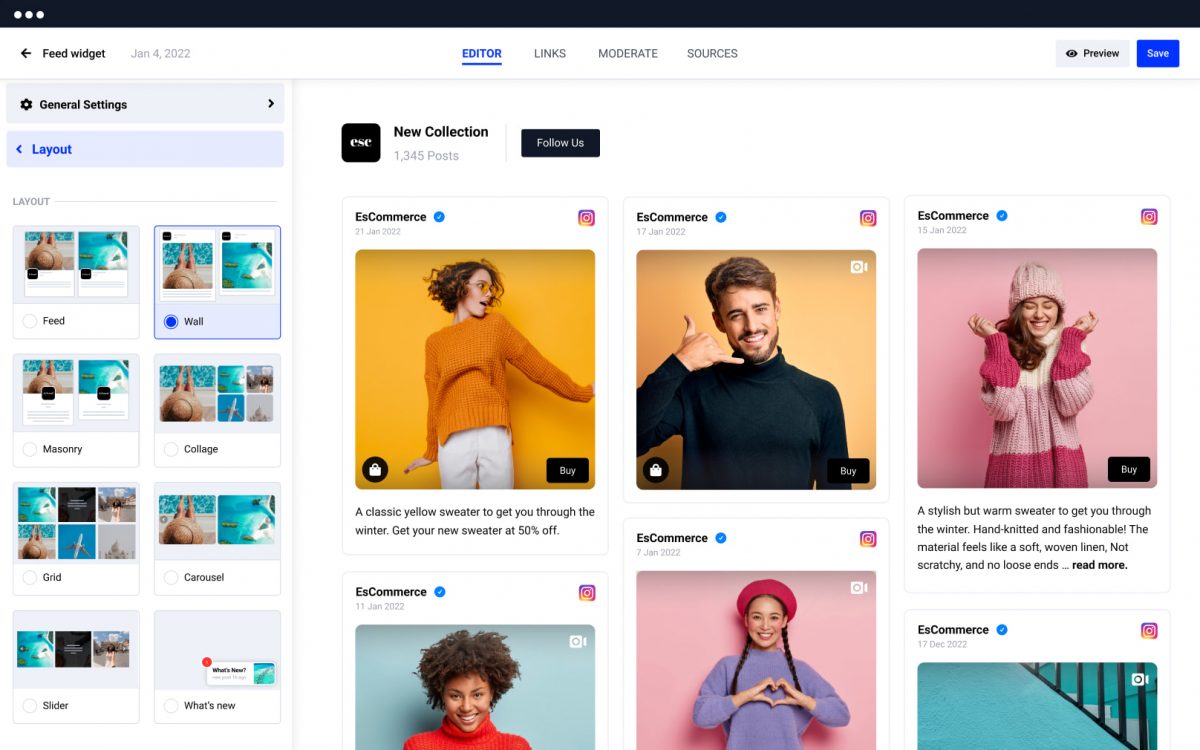Screenshot of a website interface displaying a "Feed Widget" page dated January 4th, 2022. At the top of the page, there is a black bar featuring three white circles on the left. Below this bar, the title "Feed Widget" appears in white text. An arrow pointing to the left is adjacent to navigation options: "Editor" (highlighted in blue and underlined), "Links," "Moderate," and "Sources" in black. To the right, there are a "Preview" option and a blue "Save" button.

The interface includes a section labeled "General Settings" in black and another section with "Layout" highlighted in blue. This section displays various layout options through images and titles. The first layout option features pictures resembling animals, one in blue and the others in brown. The layout is described as a feed, with options like "Wall" (blue and highlighted), "Masquerie," "Collage," "Grid," "Carousel," "Skitter," and "What's New." In "What's New," there is a small box with a red circle in the upper left corner and a small image of a bluish picture.

In the middle of the page, it mentions a "New Collection" that users can follow by clicking a black box in the upper left corner, which includes a black image with gray grading. It states "1,345 posts" and showcases several images of people. These images include a girl stretching, a man pretending to talk on a phone, a girl in a big sweater squinting her eyes, another girl smiling in a headshot, and a girl with a symbol of a heart. Additionally, there is an image resembling a staircase with a railing.